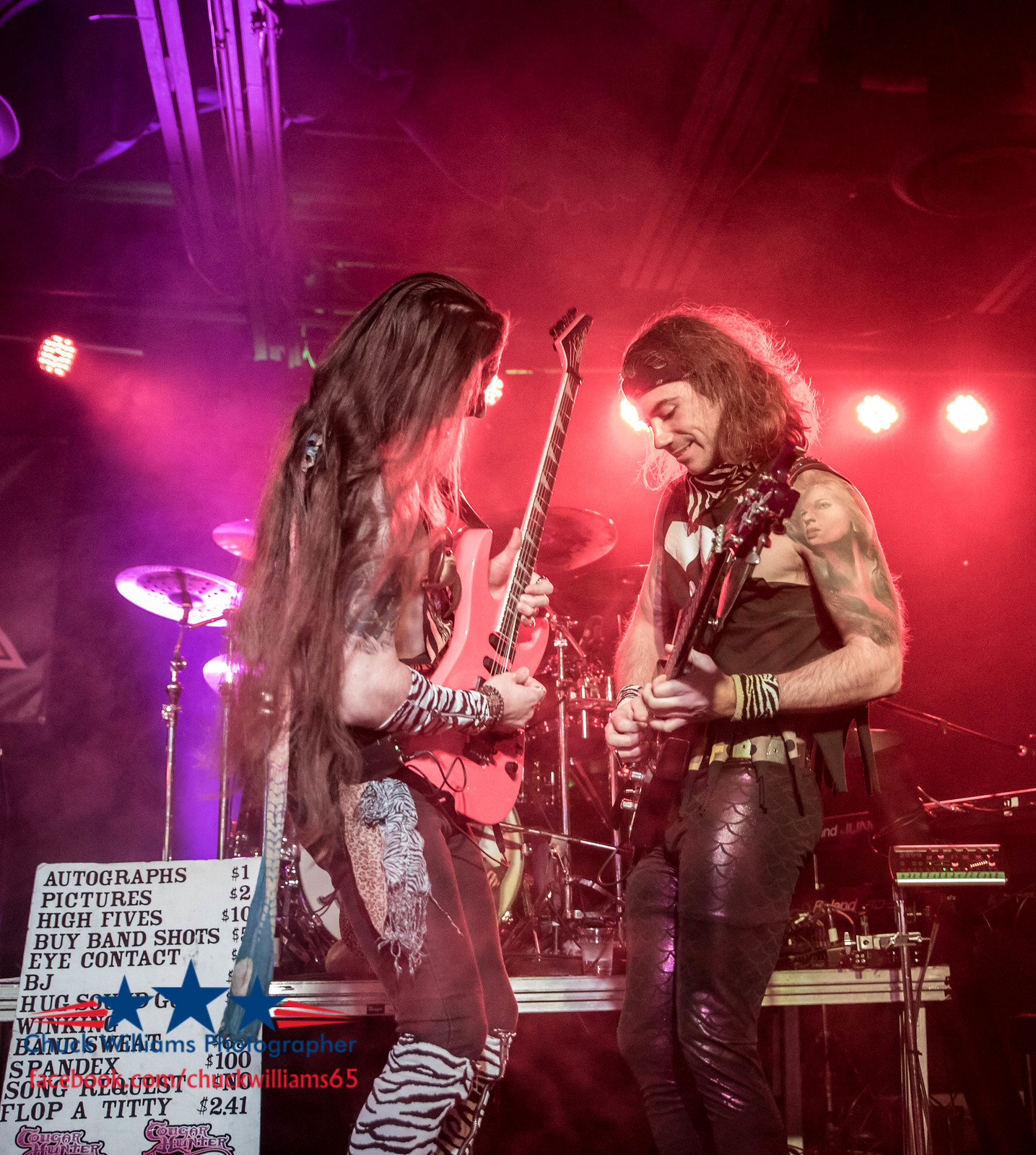This photo captures a moment at a rock concert with two electric guitarists standing center stage, facing and seemingly interacting with one another. The guitarist on the right is wearing leather pants, a cutoff t-shirt, and has long brown hair. His arms are heavily tattooed, with a notable tattoo of a woman on his left bicep. The guitarist on the left sports extremely long hair that extends below his waist, purple pants with a striking symbol on the right thigh, and white and black striped boots. He is holding a pink guitar. Both musicians project an edgy rock aesthetic, complete with the right guitarist wearing a headband or scarf.

In the background, the stage features a drum set illuminated by overhead lights, creating a dramatic atmosphere. Visible to the bottom left is a humorous merch sign listing prices for various interactions: autographs for $1, pictures for $2, high fives for $10, buying band shots for $5, and other less discernible options like eye contact and more playful entries. The sign is white with black lettering, adding a playful touch to the scene.

The overall setting is enriched with details like high beams visible in the ceiling and lights casting a glow over the stage. The varying colors in the background, including deep red and horizontal purple tones, contribute to the intense, vibrant concert environment.